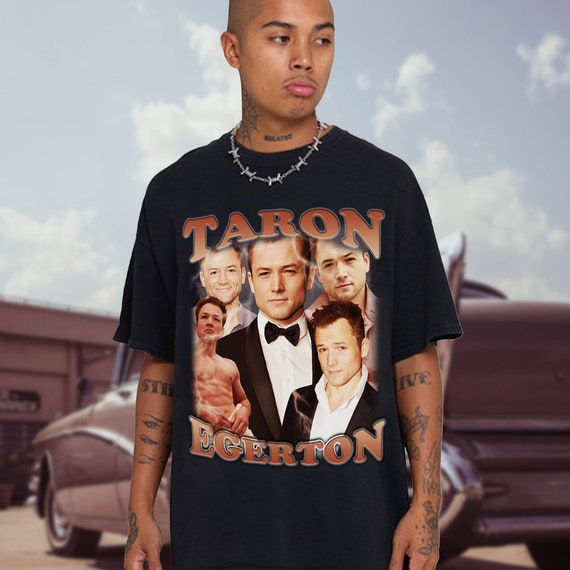This image captures a young African-American man in his late teens or early 20s, standing outdoors against a slightly blurred background. The young man has a sullen, possibly angry expression as he looks off to his left. He has an array of tattoos covering his face, neck, and arms, extending down to his hands. He wears a distinctive necklace resembling barbed wire. His black t-shirt features five images of the actor Taron Egerton, each depicting the actor in different roles and outfits.

The background showcases an older model car, possibly a vintage '57 Chevy, either in a faded pink or black and white. The car appears to be driving into a garage, hinting at the setting of a car dealership or mechanic’s shop. The sky above is blue with a few scattered clouds, adding a serene contrast to the young man's intense demeanor.